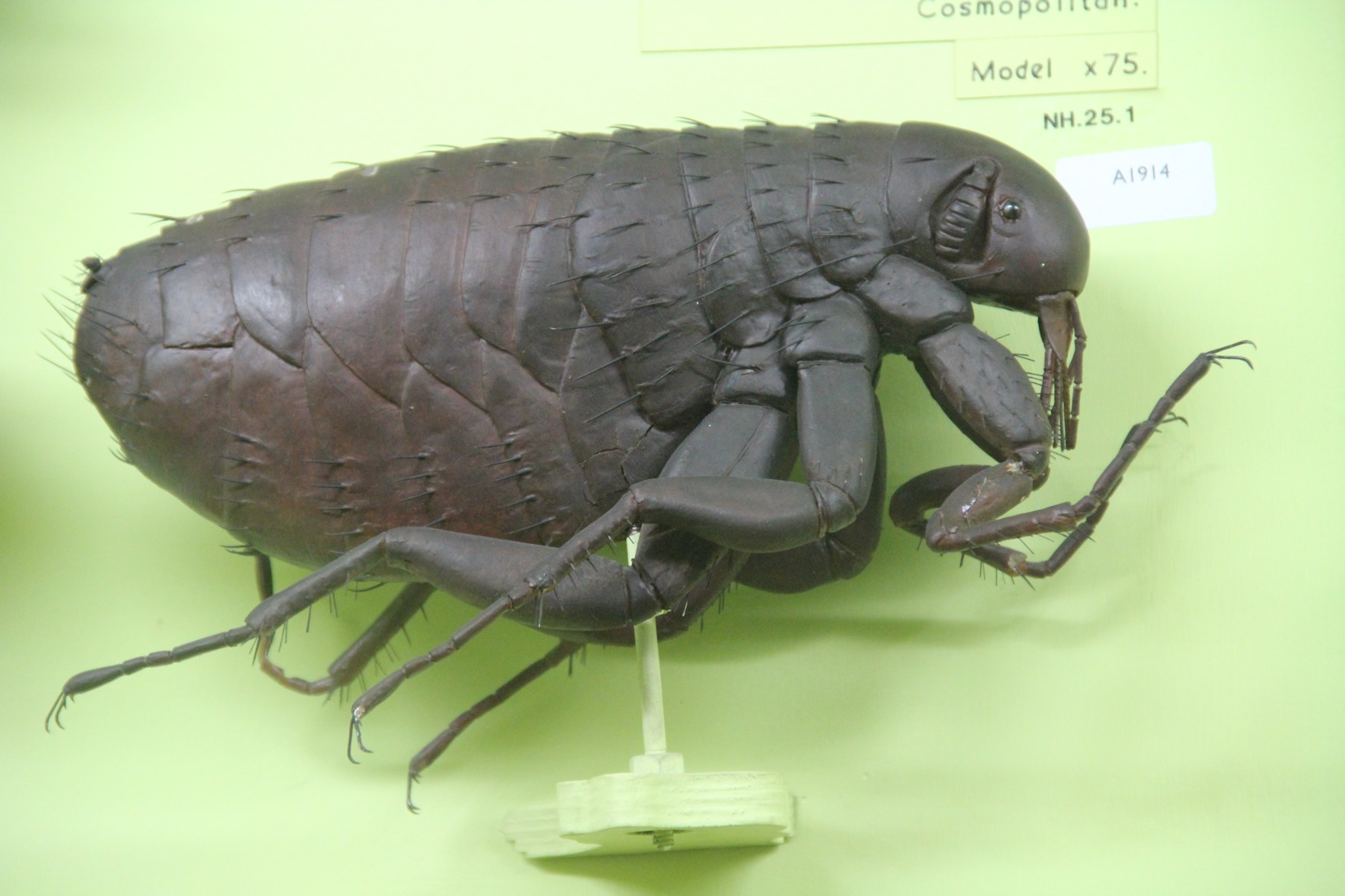The image depicts a detailed model of a plastic cockroach displayed on a small stand, set against a light green background. The cockroach is oriented with its back end on the left side of the image and its head on the right, positioned as if facing right. The model is intricately designed, featuring a segmented black body with clearly visible ridges and divisions between sections. 

The insect's anatomy includes several legs: one leg extends downwards from behind its head, bending left and up at the middle of the image before tapering back down and to the left; another similar leg is positioned in front of the first. Underneath the head, a third appendage extends slightly to the right, then curves left and downwards, and finally stretches right and upward. Fine, stringy appendages resembling mouthparts protrude from the front of the head.

The stand holding the model is visible at the bottom middle of the image, comprising a base with a pole-like section supporting the cockroach. In the background, text is partially visible, reading "composition" at the top, followed sequentially by "model," "X75," "NH 25.1," with a lighter strip below containing blue writing. The setting appears to be scientific or museum-like, suggesting the model's use for educational or display purposes.